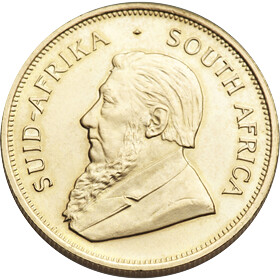This image showcases a round coin with a light beige, almost white gold appearance and some dirt around the edges. The coin features an embossed profile of an older man with slicked-back white hair, a long beard with no mustache, and wearing a suit. Surrounding the man's profile, on the left side, are the embossed words "SUID.AFRIKA" (with Africa spelled as A-F-R-I-K-A) and on the right side, "SOUTH AFRICA." The rim of the coin is dotted and the words are raised, adding to the detailed embossing.